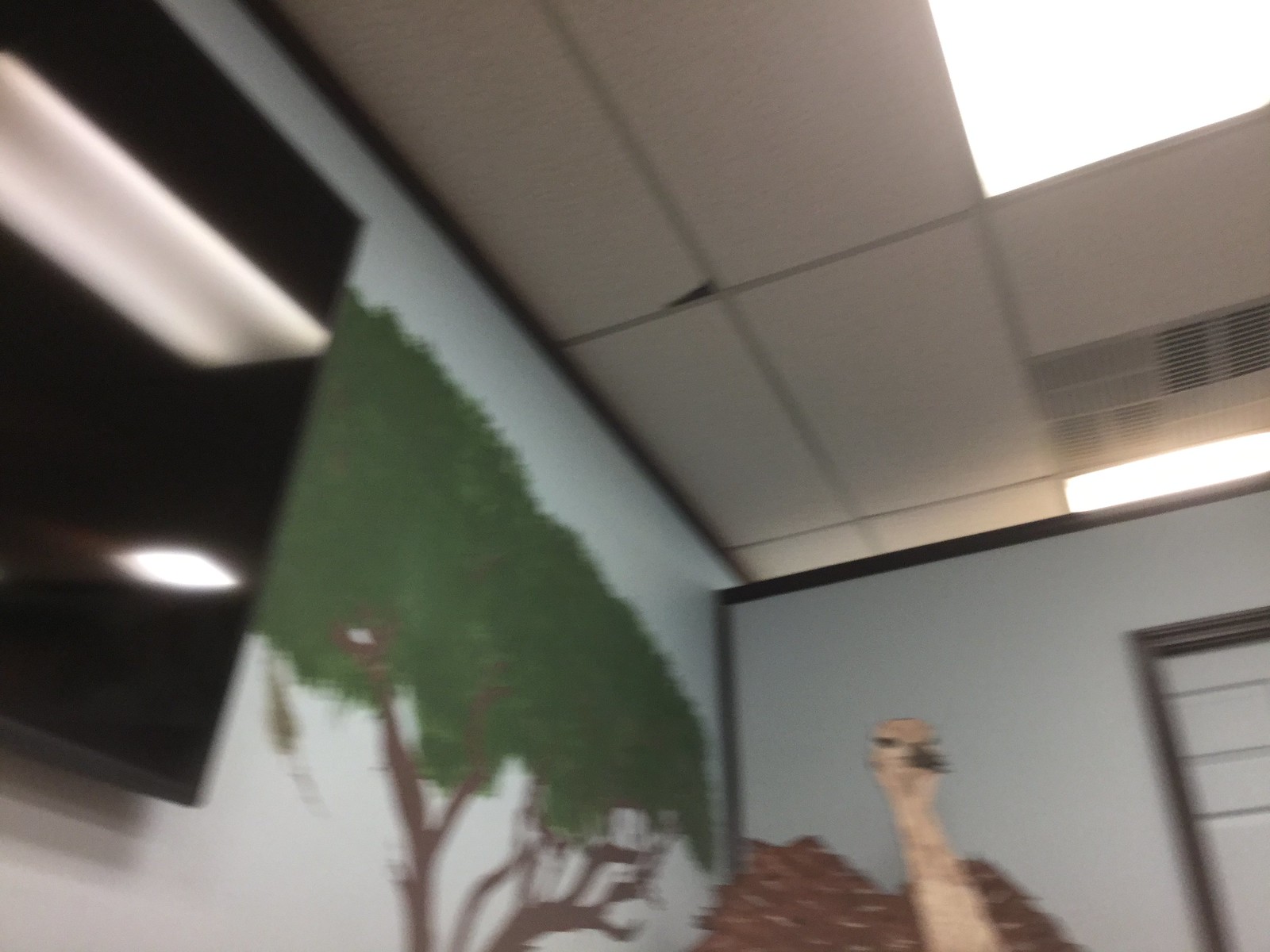This color snapshot captures an indoor scene, most likely a classroom with a glum, industrial feel. The camera is angled upwards, showcasing white acoustic ceiling tiles interspersed with fluorescent light fixtures, partially visible behind translucent panels. The room features light blue walls, one of which extends fully to the ceiling adorned with a large mural of a green deciduous tree, complete with detailed trunks and branches. The other wall only extends partway to the ceiling, outlined with wooden trim, and decorated with a mural of a detailed ostrich—its black eyes, pinkish neck, and brown tail feathers are prominently depicted. Adding to the room's detail, a wall-mounted, black TV appears on the left side, turned off but reflecting the glow of the fluorescent lighting. The bottom right corner of the image features additional wood trim around what seems to be a door, enhancing the room’s structured layout.